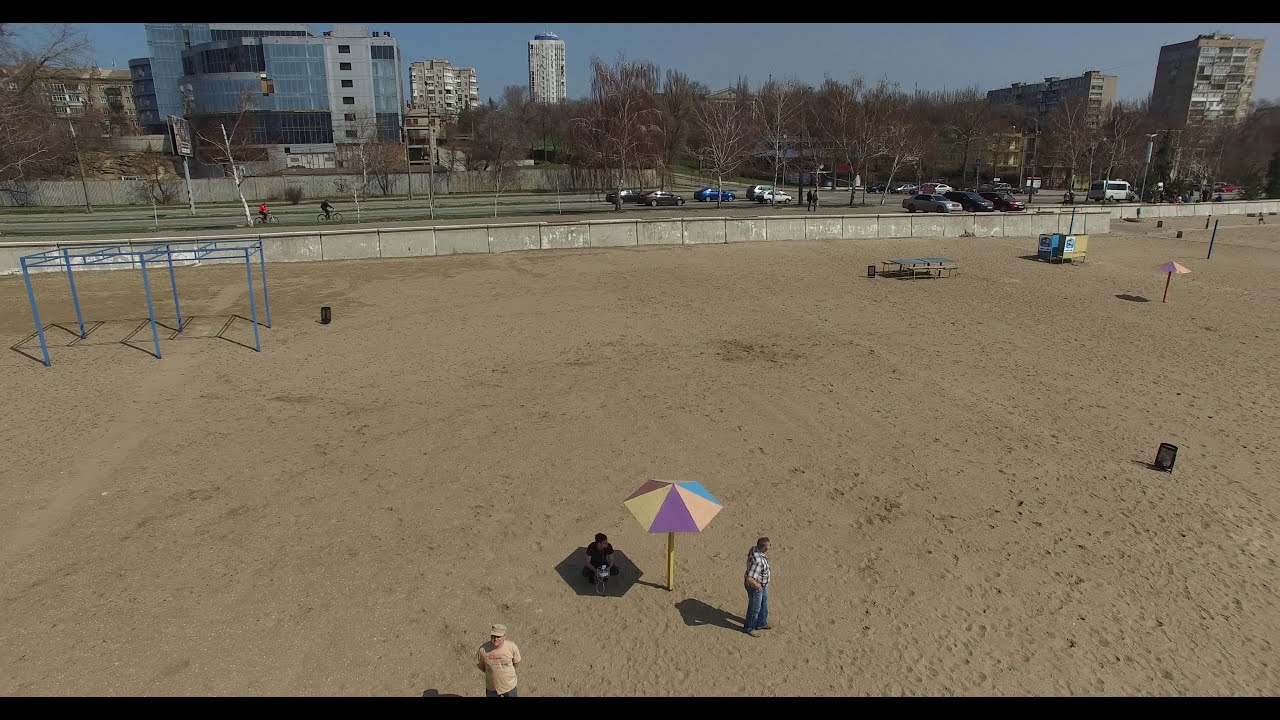The image showcases an elevated, overhead view of a beach area devoid of visible water but abundant in sand. In the foreground, a multicolored umbrella in shades of blue, yellow, and purple stands prominently, providing shade to a man with a dog. Nearby, a man in an orange t-shirt with a beige cap and another man in a plaid shirt and jeans linger close by. The area seems sparsely populated, hinting at cooler weather, which is further suggested by the leafless trees visible in the background.

The sandy expanse extends back to a low cement beach wall, beyond which lies a two-lane road with parked cars and a couple of cyclists passing by. To the left of the sand, there’s a metal structure with six legs, likely an exercise bar for pull-ups. Towering over the scene in the background are several buildings, including a couple of mid-rises and a distant skyscraper, all set against a clear, bright blue sky indicating a sunny daytime setting.